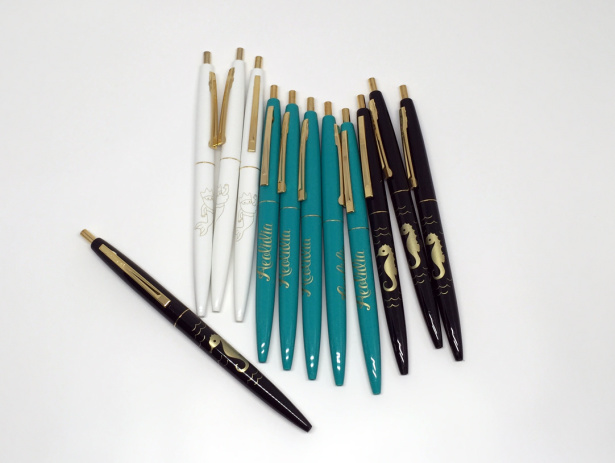This detailed color photograph, taken indoors under artificial light, captures a collection of retractable ballpoint pens artfully laid out on a white surface. The square image, which appears to be staged, exhibits no definitive borders and features a pens organized in a jagged line. The pens are presented in three distinct colors: black, turquoise, and white, each adorned with gold-colored accents.

On the left side of the image lies a single black pen angled towards the upper left corner. This pen, like three others positioned on the far right, features a gold seahorse design. Centrally placed are five turquoise pens with gold accents and cursive gold writing that remains illegible due to the twist of the pens. In between these, three white pens bear intricate gold designs of a regal merman with a crown and a prominent beard.

Each pen showcases a uniform design: a solid two-section barrel with a visible brass ring at the midpoint, a brass clicker at the top, and a brass clip partially running down the side. The arrangement and detailed embellishments highlight the uniqueness of each pen while maintaining a cohesive aesthetic.